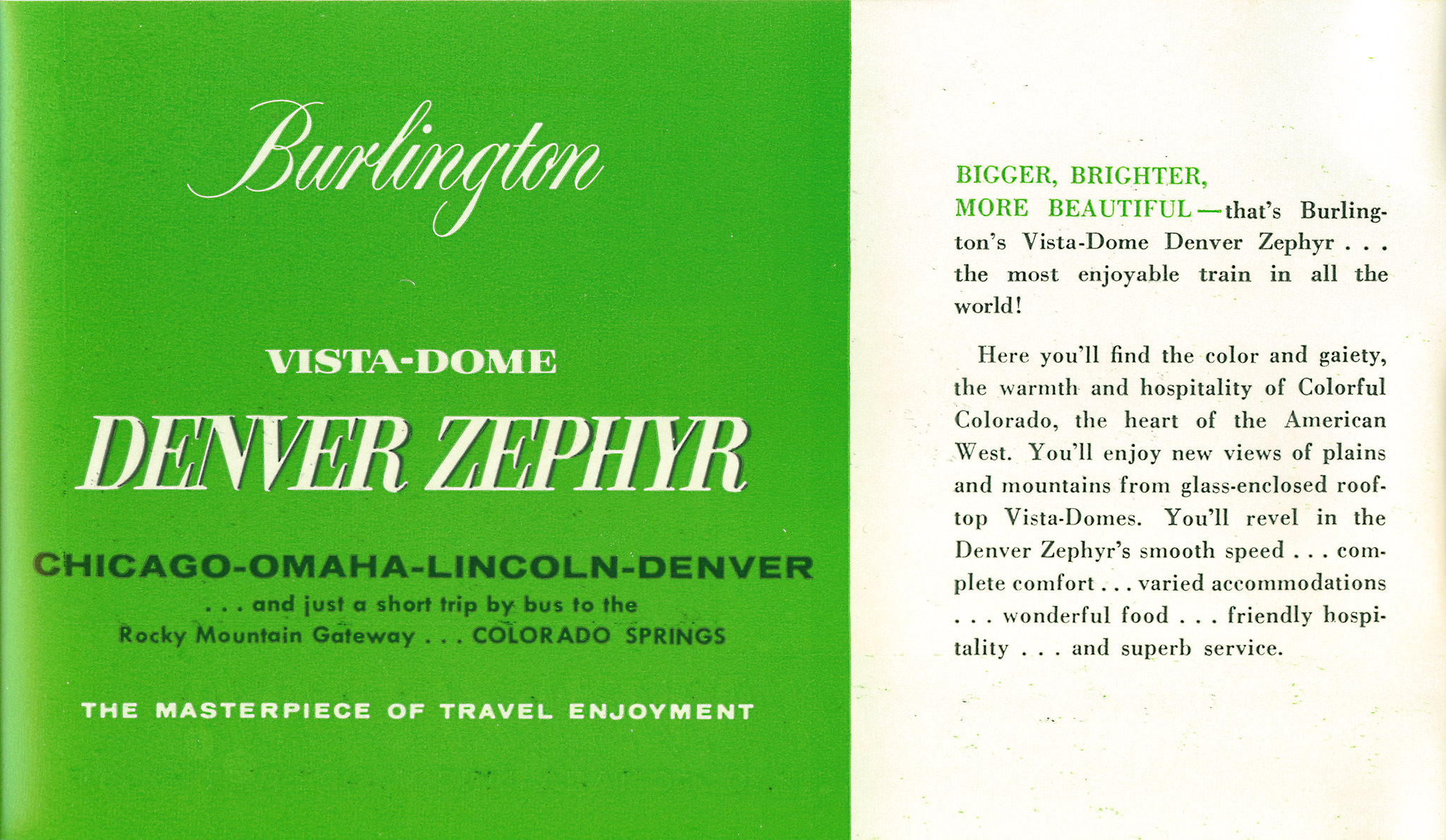The image is a detailed advertisement for the Burlington Vista-Dome Denver-Zephyr. This print piece is split into two panels: the left panel has a green background with white and black text, while the right panel features a white background with green and black text. At the top of the green panel, "Burlington" is elegantly written in cursive, followed by "VISTA-DOME" and "DENVER-ZEPHYR" in all caps. Below this, a series of black text lists the destinations, reading "Chicago, Omaha, Lincoln, Denver," and mentions "just a short trip by bus to the Rocky Mountain Gateway, Colorado Springs," describing it as a "masterpiece of travel enjoyment." On the far right of the image, a headline reads, "Bigger, Brighter, More Beautiful," with additional black text beneath it emphasizing the unmatched pleasure of traveling on Burlington's Vista-Dome, Denver-Zephyr, hailed as the most enjoyable train in the world. This beautifully designed piece functions as an enticing advertisement for an exceptional train travel experience.